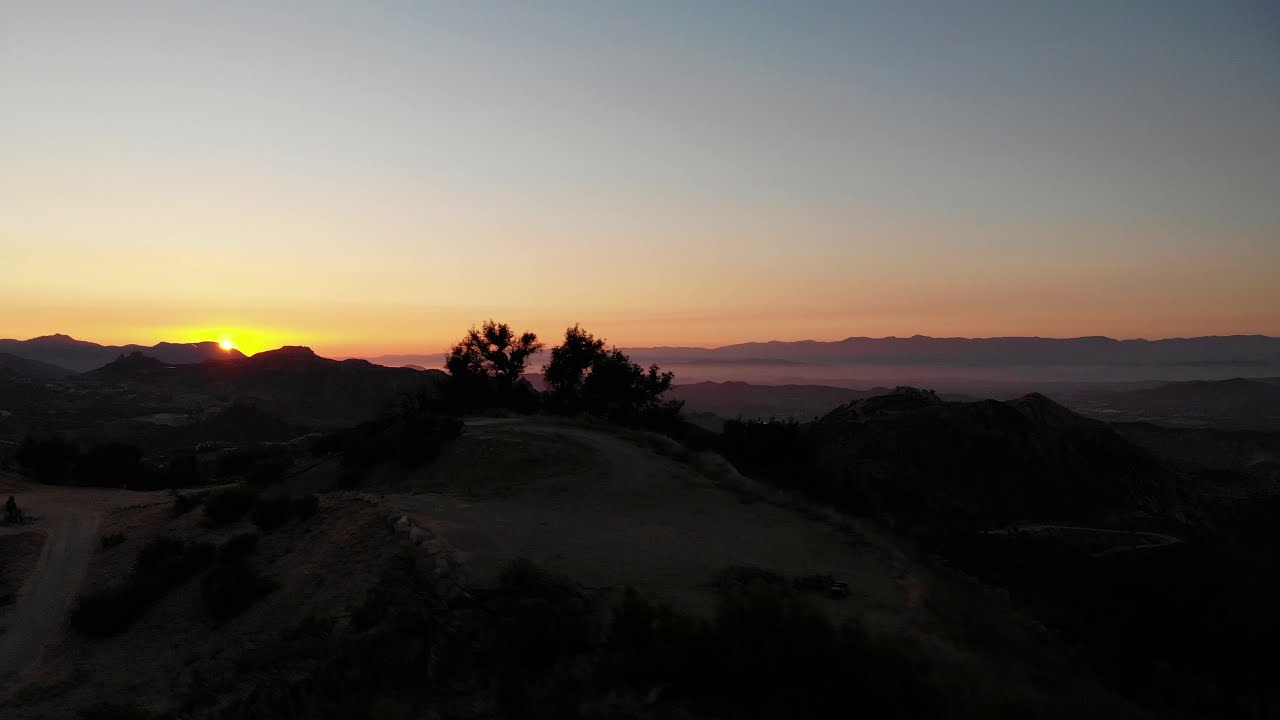This color photograph captures a breathtaking aerial view of a mountainous landscape at sunset. The image, taken from near or at the top of a mountain range, showcases a striking scene where the bottom half is dominated by the silhouettes of mountains and sparse trees against a brilliantly colored sky. A winding road is visible in the lower left side, descending from a relatively flat mountaintop area that looks like an open parking spot or a small plateau. The sun, nestled low on the horizon on the left side of the image, bathes the sky in a stunning gradient of yellows, oranges, and purples, ultimately fading into blue towards the top. The photograph, free of clouds, also hints at a hazy valley below, where a faint silhouette of a body of water can be seen amidst the fog that lingers between the distant mountain ridges. The realism and naturalistic style of the photograph make it a captivating and serene depiction of nature at its most picturesque moment.